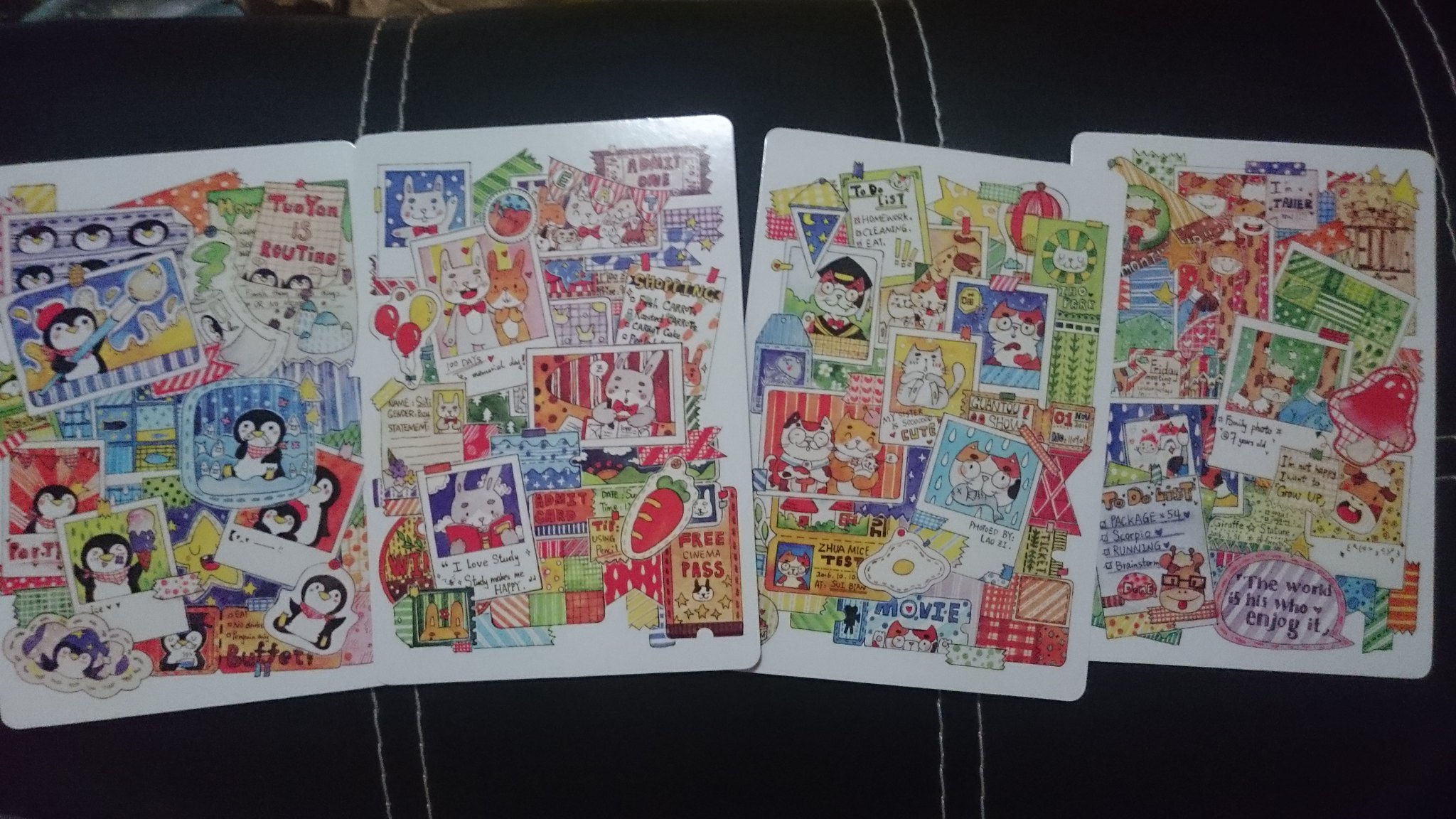The image depicts four colorful cards, each with vibrant illustrations and playful designs, laid out on a surface that appears to be black leather with white stitching, possibly a couch. The cards, approximately four and a half inches wide by three inches tall, are arranged closely together, emphasizing their artistic details. 

The first card features charming illustrations of penguins enjoying ice cream and bears the text "To you, it's routine." The second and third cards are adorned with various expressive cats, each showcasing different amusing poses and facial expressions. The fourth card stands out with a whimsical design that includes a mushroom and what appears to be dogs, suggesting a playful, dog-themed motif. These cards, with their eye-catching colors and child-friendly imagery, seem to be intended for young children, around three years old, offering them delightful and engaging illustrations to enjoy.